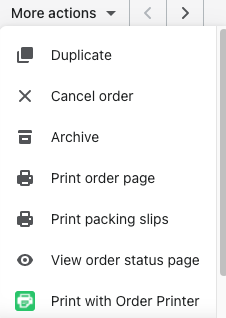A cropped screenshot of a webpage reveals a "More Actions" dropdown menu commonly found on platforms related to shipping and packaging. The menu includes several options: "Duplicate," "Cancel Order," "Archive," "Print Order Page," "Print Packing Slips," "View Order Status Page," and "Print with Order Printer." Each option is accompanied by a distinct icon: "Duplicate" displays two copies of a form, "Cancel Order" shows an X, "Archive" features a storage box, "Print Order Page" and "Print Packing Slips" have icons typical for printing, and "View Order Status Page" includes an eyeball. Notably, while most icons are black and white, the "Print with Order Printer" option is highlighted with a green icon depicting a white printer. Additionally, there's a forward button, suggesting that this view is part of a larger interface. The overall design includes a white background with black text, enhancing readability. Though the exact website name isn't visible, the context strongly implies that the site is related to management of shipping and packaging orders.